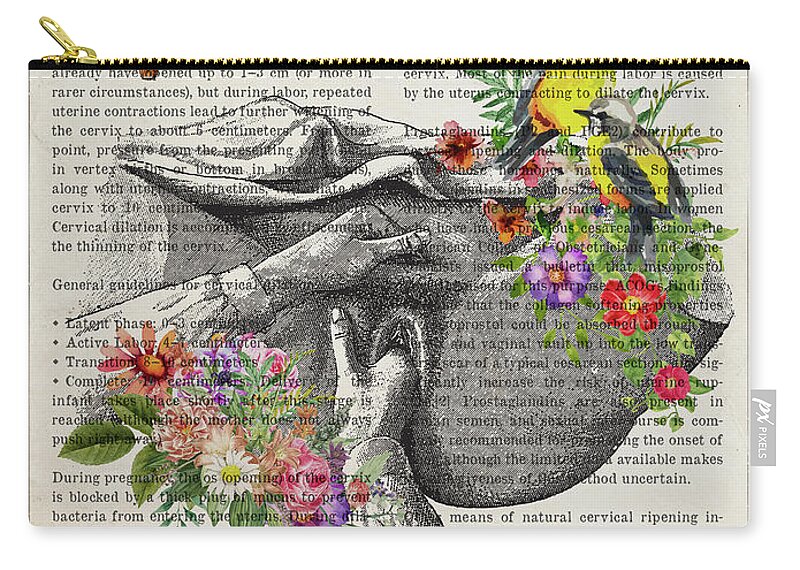The image depicts a small, greyish-beige coin purse with a gold zip and a black felt line directly below the zipper, which is positioned on the left side. The coin purse features an intricate design that includes detailed text outlining guidelines for a cervical examination, such as information about the uterus dilating and cervix ripening. Complementing the textual elements, the purse showcases a vivid array of flowers in various colors (green, orange, white, purple, pink, red, and blue) situated in the bottom left and top right corners. Additionally, the artwork includes two birds with yellow bodies, black wings, black beaks, and brown and white heads. A striking, hand-drawn image in the background highlights a doctor performing a vaginal exam, emphasizing the medical context. Finally, a tag on the bottom right corner of the purse bears the cursive inscription "PX" followed by the word "PIXELS" in all capital letters.